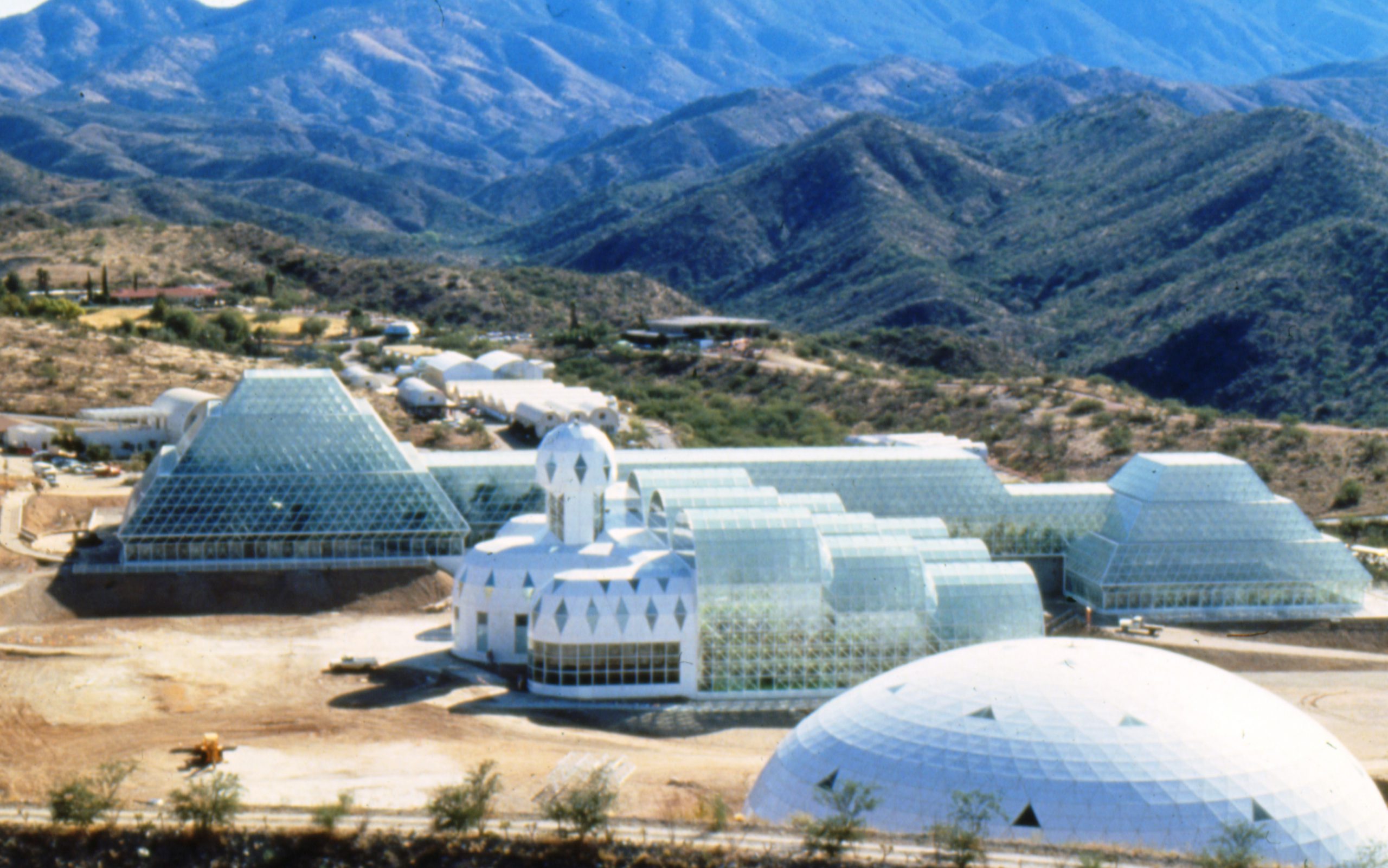Amidst a rugged, scrub-filled hillside with exposed sandy areas, an intricate collection of buildings stands prominently against a backdrop of distant, lush green mountains and rolling hills. The foreground reveals a trio of significant architectural structures, each with distinct features. At the bottom of the image, a striking white dome composed of triangular shapes and accented with black triangles commands attention. Just beyond, a complex structure with a combination of white walls and translucent glass arranged in cascading semicircles adds a modern flair to the scenery. To the far left, a gleaming glass pyramid captures and reflects the sunlight, creating an ethereal effect. On the far right, a layered rectangular block structure balances the composition. The dry, brown and dirt-covered ground, interspersed with young, thin trees, contrasts with the verdant mountains, creating a vivid scene of juxtaposed natural and architectural beauty.